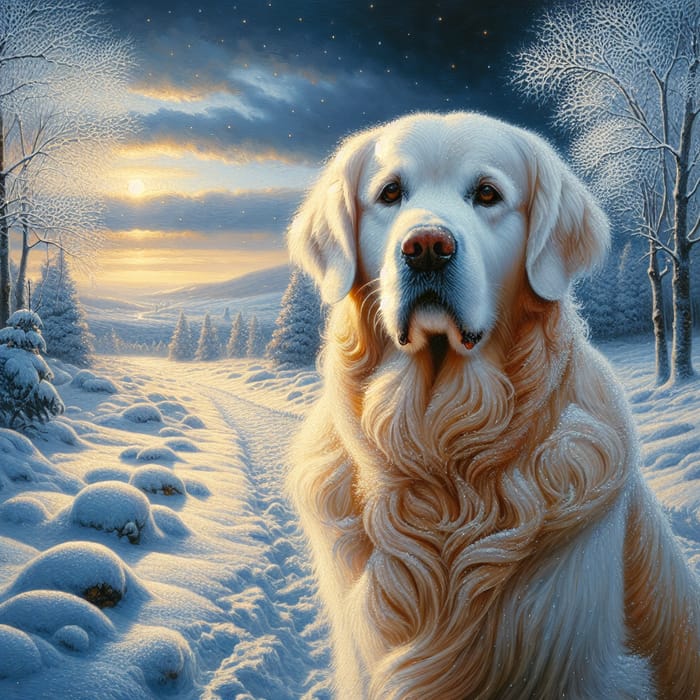This is a digital artwork depicting a serene winter scene featuring an elegant golden retriever. The dog, a white-faced, light cream-colored retriever with a shaggy mane of golden curls, sits prominently in the right foreground, filling much of the frame from the chest upward. Its floppy ears hang by the sides of its head, and it gazes with brown eyes past the viewer, its pinkish-red nose standing out against its white and golden fur.

The landscape is bathed in the warm, pale yellow light of a setting sun, which glows in the distant sky, partially obscured by streaks of dark blue and gray clouds. Snow blankets the entire scene, covering a trail that winds through the snowy woodland, flanked by towering pine trees and various bushes all encrusted in snow. The trees, some shaped like traditional Christmas trees, and others tall and barren with snow-dusted branches, frame the scene, adding to the tranquil atmosphere. Far in the background, the snow-covered mountain range extends across the horizon, completing this picturesque winter tableau.